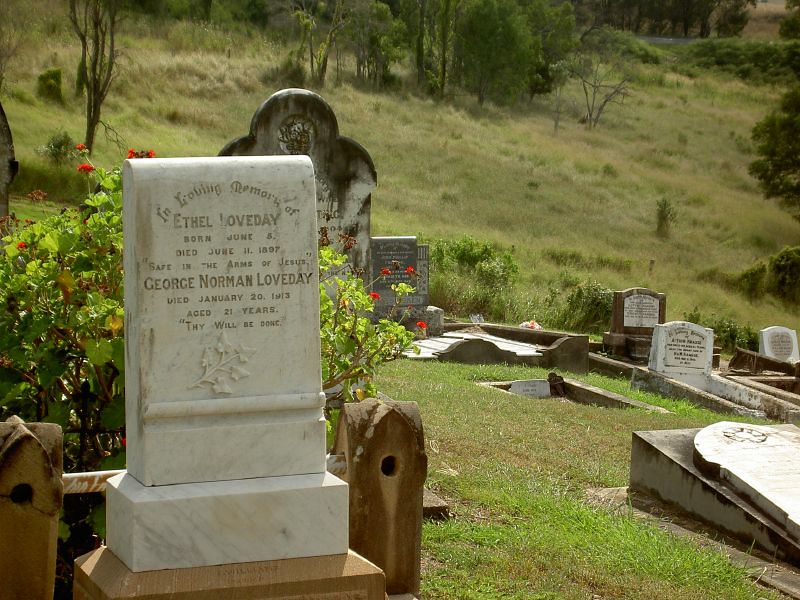The daytime photograph captures a tranquil cemetery scene, featuring a prominent white marble headstone positioned on the left side of the image. The headstone reads, in cursive script, "In loving memory of Ethel Loveday, born June 5th, died June 11th, 1897. Safe in the arms of Jesus." Below this, it commemorates "George Norman Loveday, died January 20th, 1913, age 21 years. Thy will be done," and includes an engraving of a leaf or flower. The headstone, square with rounded edges, stands in the foreground, surrounded by various smaller and larger grave markers. In the background, grassy hills and some vegetation can be seen extending towards the horizon, adding a touch of natural serenity to the scene. A large bush with red flowers grows nearby, contributing to the peaceful ambiance of this historic resting place.